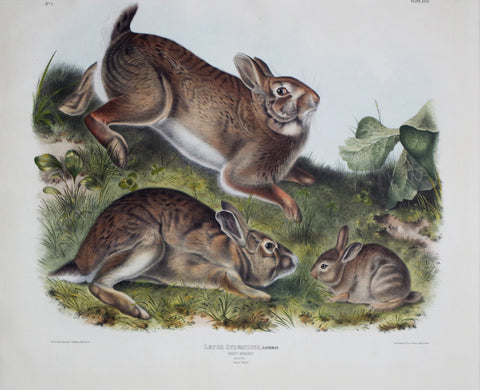The detailed drawing features three rabbits set against the backdrop of grassy terrain, complete with green cabbage leaves and scattered small rocks. At the topmost part of the hill, a large adult rabbit stands with its ears pulled back and nose up, appearing alert. Below, a medium-sized rabbit lies on its side, with outstretched legs and ears also laid back. Nose-to-nose with this reclining rabbit is a tiny bunny, characterized by its straight, upright ears and a small tail. All three rabbits sport a healthy appearance, with brown fur adorned with black spots, darker tails, and white underbellies. Whiskers are also visible on the rabbits, adding to their lifelike depiction.